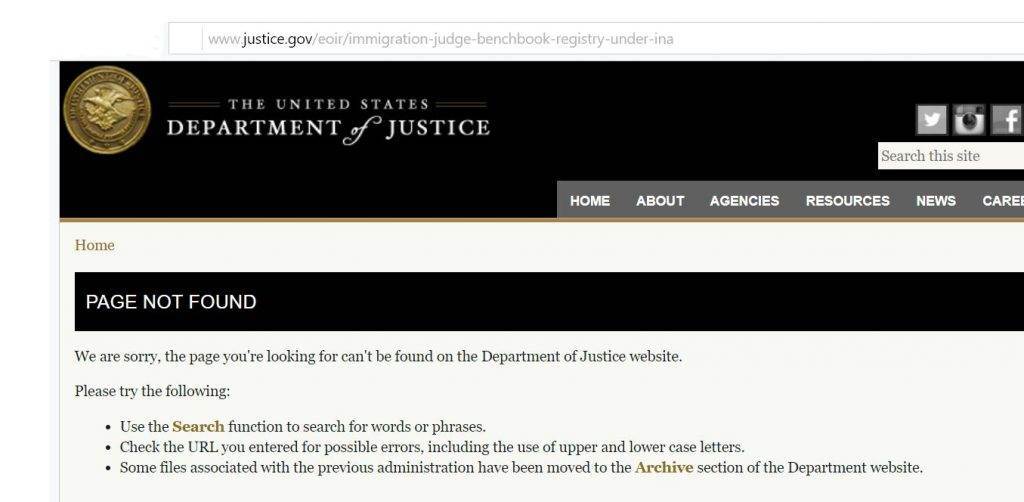The image depicts a partially captured webpage from the official website of the United States Department of Justice, accessible at www.justice.gov. At the top of the webpage is the address bar, displaying the URL, followed by the department's emblem on the left side. The gold emblem prominently features an eagle at its center, encircled by laurel branches and inscribed with the words "The United States Department of Justice." The word "of" in the inscription is in a cursive and italicized font.

To the right of the emblem is a horizontal navigation menu set against a gray background. The menu includes tabs labeled "Home," "About," "Agency Resources," "News," and "Careers," though the "Careers" tab appears to be slightly cut off. Directly above this navigation menu is a search bar accompanied by icons for social media platforms: Facebook, Instagram, and Twitter.

Below the navigation menu, the text "Home" is displayed on the left-hand side, followed by a prominent black banner stating "Page Not Found." The message beneath reads, "We are sorry, the page you're looking for can't be found on the Department of Justice website." The text then suggests possible actions in a bulleted list, with the first suggestion highlighting "search" in an orange color for emphasis.